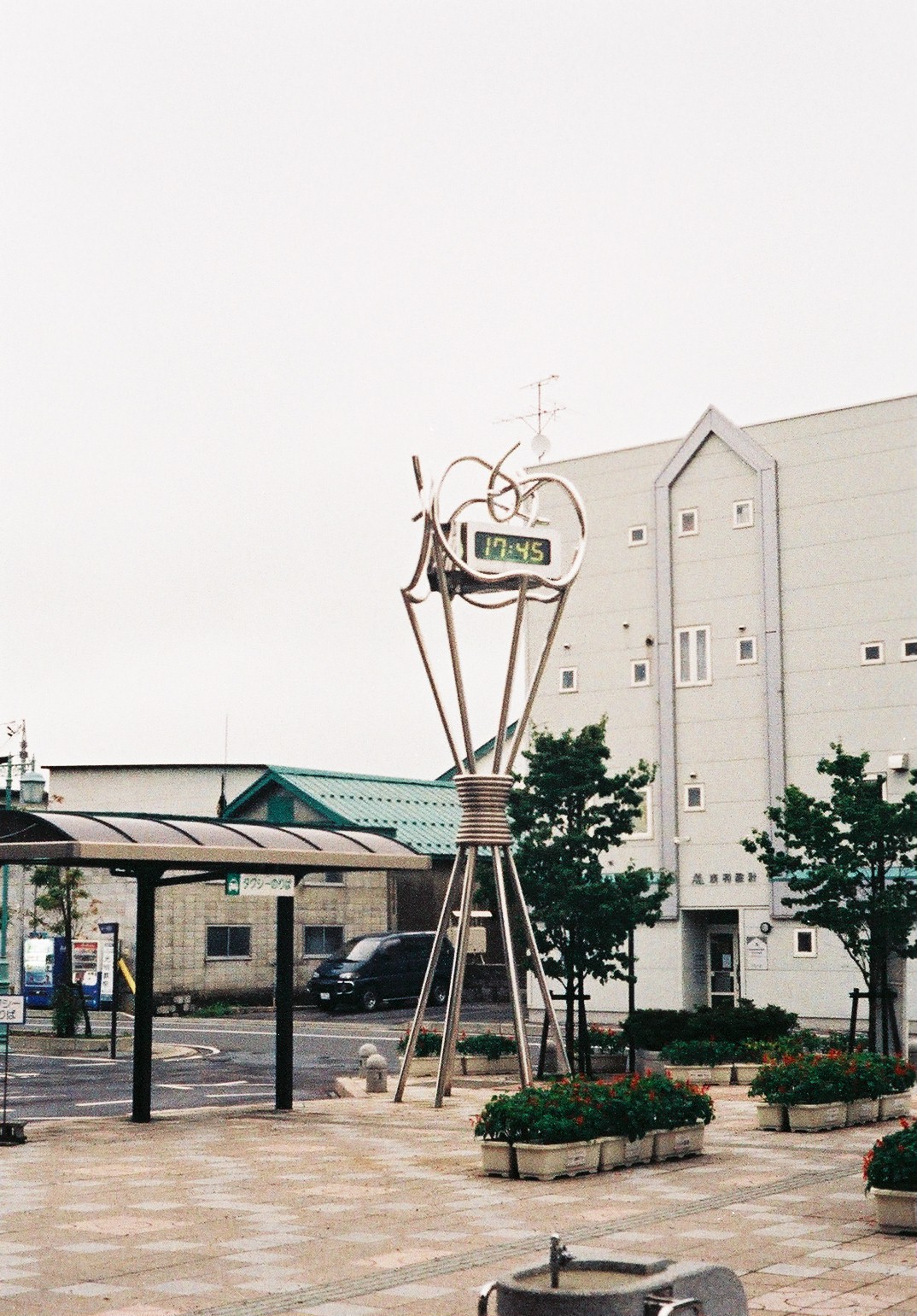The image captures an urban cityscape, centered around a unique clock structure. This impressive clock, resembling an elongated hourglass, features a tower made of sleek, silver steel pipes. The tower's design includes a series of circular pipes intertwined in the middle, flanked by an upward extension that culminates in an apple-like shape formed by gracefully curved steel bars. In the heart of this intricate structure is a digital clock display, showing the time as 17:45, illuminated in a vibrant light green hue. Surrounding the clock, bright lights accentuate its modern design.

To the right of the clock, a large building looms in the background, adding to the city’s architectural depth. On the left, a smaller building, seemingly a store, contributes to the diverse skyline. Adjacent to the clock on the left side is a bus stop, offering a convenient resting place for commuters. The scene is grounded by a light gray concrete sidewalk that stretches beneath the clock. Adding a touch of natural beauty, various bushes and plants are arranged in rectangular compartments along the sidewalk, seamlessly integrating greenery into the urban environment.